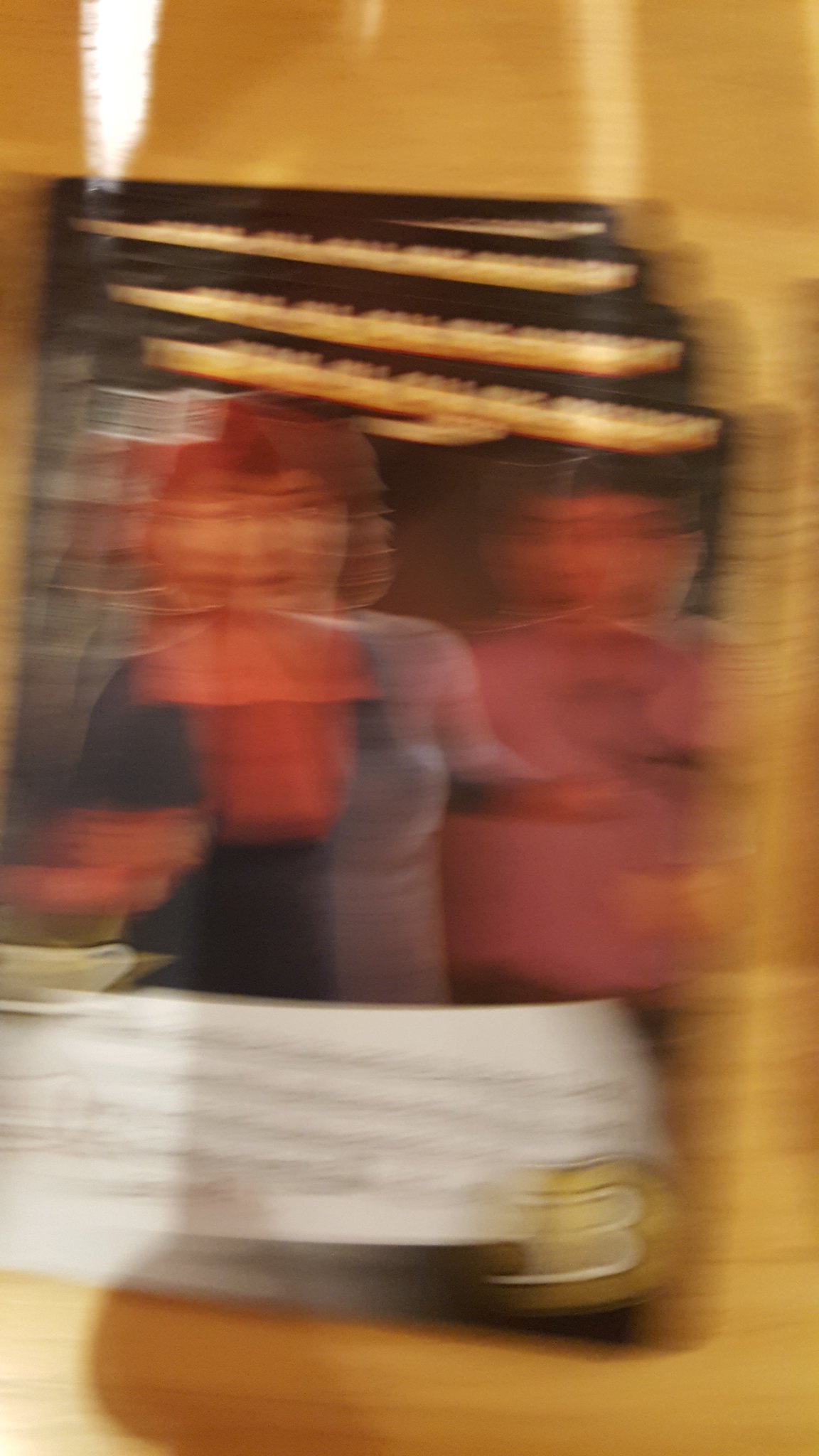In this extremely blurry image, it appears to depict multiple baseball card-like objects laid out on a glossy tabletop. Each card features cartoon-like illustrations of people, some in motion, rather than real-life photographs. Among these figures, one appears to be a man and possibly two women, distinguished by their attire—one in a pink shirt and another in a blue shirt. There is a white blurb of text positioned at the bottom of each card, though its content is indiscernible due to the blurriness of the image. The overall scene is difficult to interpret with complete accuracy because of the lack of clarity, but it gives the impression of an assortment of collectible cards displaying animated characters.